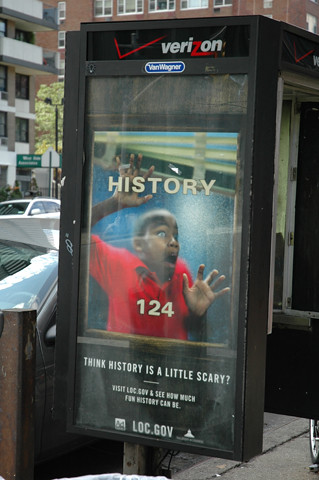The photograph depicts a sidewalk scene featuring a structure resembling a phone booth, though it is actually a Verizon advertisement display. The booth-like structure has a black top with the Verizon logo prominently displayed in white. Just below the logo, there is a bold blue banner labeled "Von Wagner." The main display of the advertisement features a movie poster that showcases a young boy in a bright red shirt with a shocked expression. His right hand is pressed flat against the poster, and his left hand is at shoulder height. Across the poster, the word "history" is printed in white, with the number 124 in front of his chest. The poster includes a caption at the bottom stating, "think history is a little scary." Below this message is a smaller text, partially readable, directing to the website loc.gov. 

In the background, you can see several elements of an urban environment. There are brick apartment buildings with white-barrier balconies and multiple windows. One of the buildings is partially obscured by the advertisement display. There are also street lights, a couple of green trees, and various vehicles, including a partially visible white car and a small silver car. The scene is well-lit, suggesting it was captured during the daytime. The concrete sidewalk and a metal pole are also noticeable in the foreground.